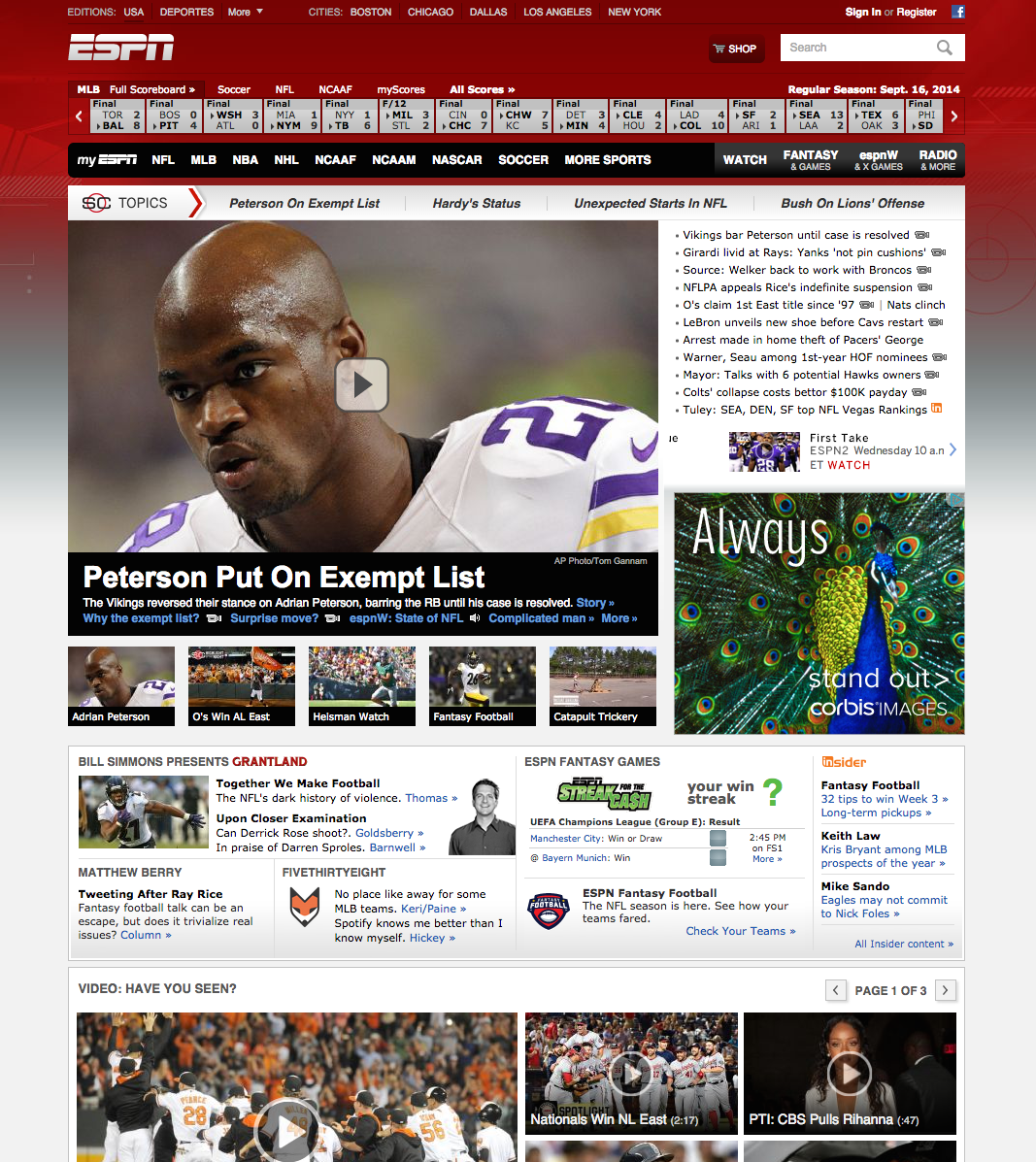The image features a gradient background transitioning from red at the top to gray, then to a lighter gray towards the bottom. At the top-center, there are white text elements that are difficult to read. The right-hand side displays a Facebook symbol. The upper-left corner features the ESPN logo. Below this logo, a darker red rectangle with a shopping cart icon and the word "Shop" in white is visible. Adjacent to it, a white rectangle with the word "Search" on the left and a magnifying glass symbol on the right is present. Another dark red rectangle containing unreadable text follows, with additional text underneath.

Below this section, there is a series of gray rectangles possibly listing various sports scores, although they are unclear. A black rectangle on the right displays "My ESPN" and suggests categories like NFL, MLB, NBA, NHL, NCAAF, NCAAM, NASCAR, and soccer, among others. Directly following these categories are the options "Watch," "Fantasy," an unreadable third item, and "Radio."

A white bar runs across the page, featuring the letters "SC" partially covered by a red circle, accompanied by the word "Topics" and an arrow pointing to the right. On the left-hand side, an image of a football player is displayed, within which a white triangle pointing right indicates a video. Below this video component, a black rectangle contains the text "Peterson put on exempt list" and additional white and blue text underneath. Smaller images are situated below this section.

To the right of the video area, there is a light gray square with substantial text and a small, indistinct picture at the bottom. Beneath this section, an image of a peacock with the text "Always stand out" and an arrow pointing right linked to Corbis Images.

Returning to the left-hand side, the next element is another black rectangle with further text and blue highlights, plus smaller pictures below. A gray rectangle showcases another image of a different football player, text in black and blue, and some unreadable elements. Nearby, a fox-like symbol is present along with a head-and-shoulders image of a man.

To the immediate right, there is a section advertising "ESPN Fantasy Games" with a green logo, text about "your win streak," and further writing in orange, black, and blue. Another logo appears red and black with similar text styling.

Towards the bottom, a white rectangle with the heading "Videos you have seen" appears, featuring navigation arrows in gray squares indicating page numbers and further thumbnail images marked with a video symbol.